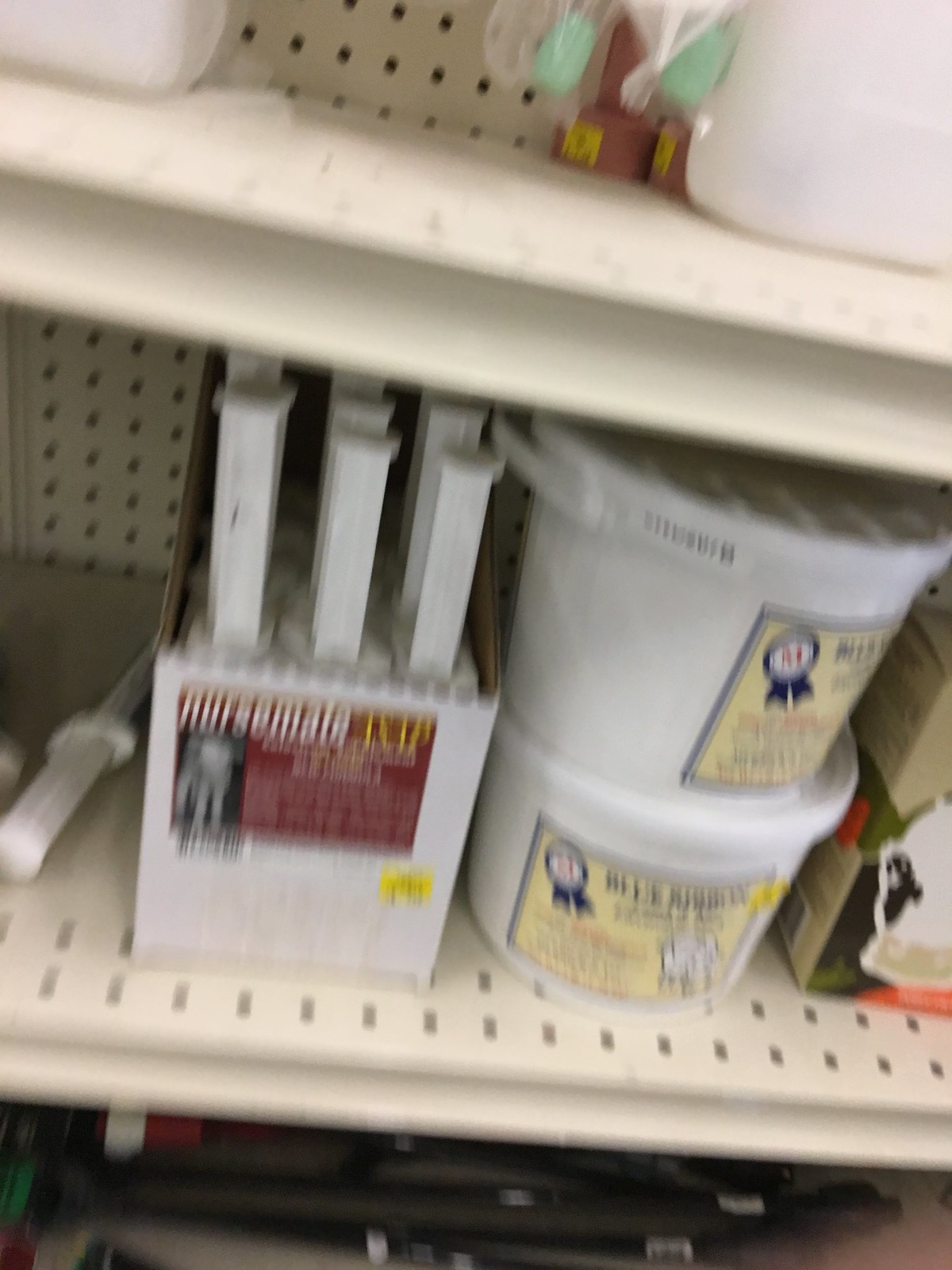This image, taken in a store—likely a hardware store—depicts three slightly blurry metal shelves with small holes, characteristic of metal shelving units. The top shelf houses white containers beside circular objects featuring yellow stickers, possibly bricks. The middle shelf contains two stacked white plastic tubs adorned with a cream-colored label depicting a blue ribbon and partially legible text suggesting a product, possibly named "blue ribbon." Adjacent to these tubs is a white box with a dark red label reading "Nurse Mate" in white, containing several long, white cartridge-like objects that are difficult to identify but could be thermometers. The bottom shelf, only partially visible, holds an indiscernible black and metal object, adding to the mysterious assortment in this slightly blurred snapshot.